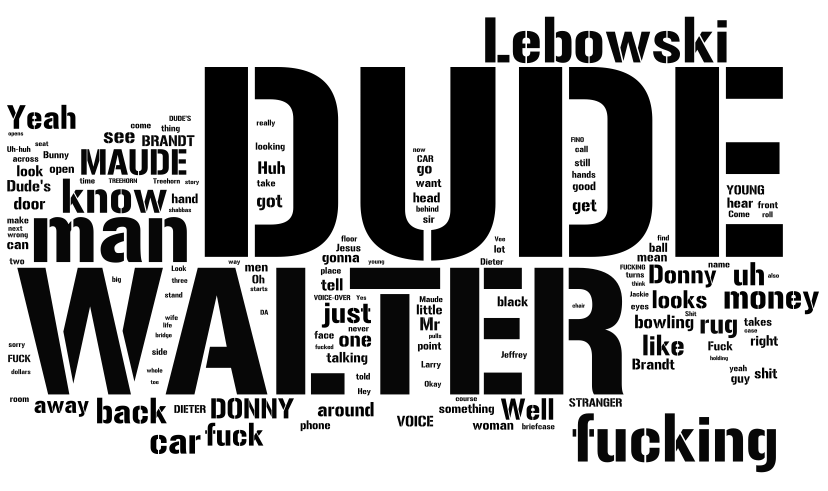The image is a visually striking word cloud set against a white background, composed entirely of text related to "The Big Lebowski." In this collage-style graphic, words vary in size based on their frequency within the context of the movie. Dominant terms such as "Lebowski," "dude," and "Walter" stand out prominently, while smaller words like "yow," "mod," "no man," "Donnie," "fucking," "money," "bowling," and "rug" create a scattered yet cohesive arrangement. The overall design lacks any particular centered focus, further emphasizing its collage nature. The black text on a white background ensures clarity, allowing for an easy visual analysis of word prominence and connections.